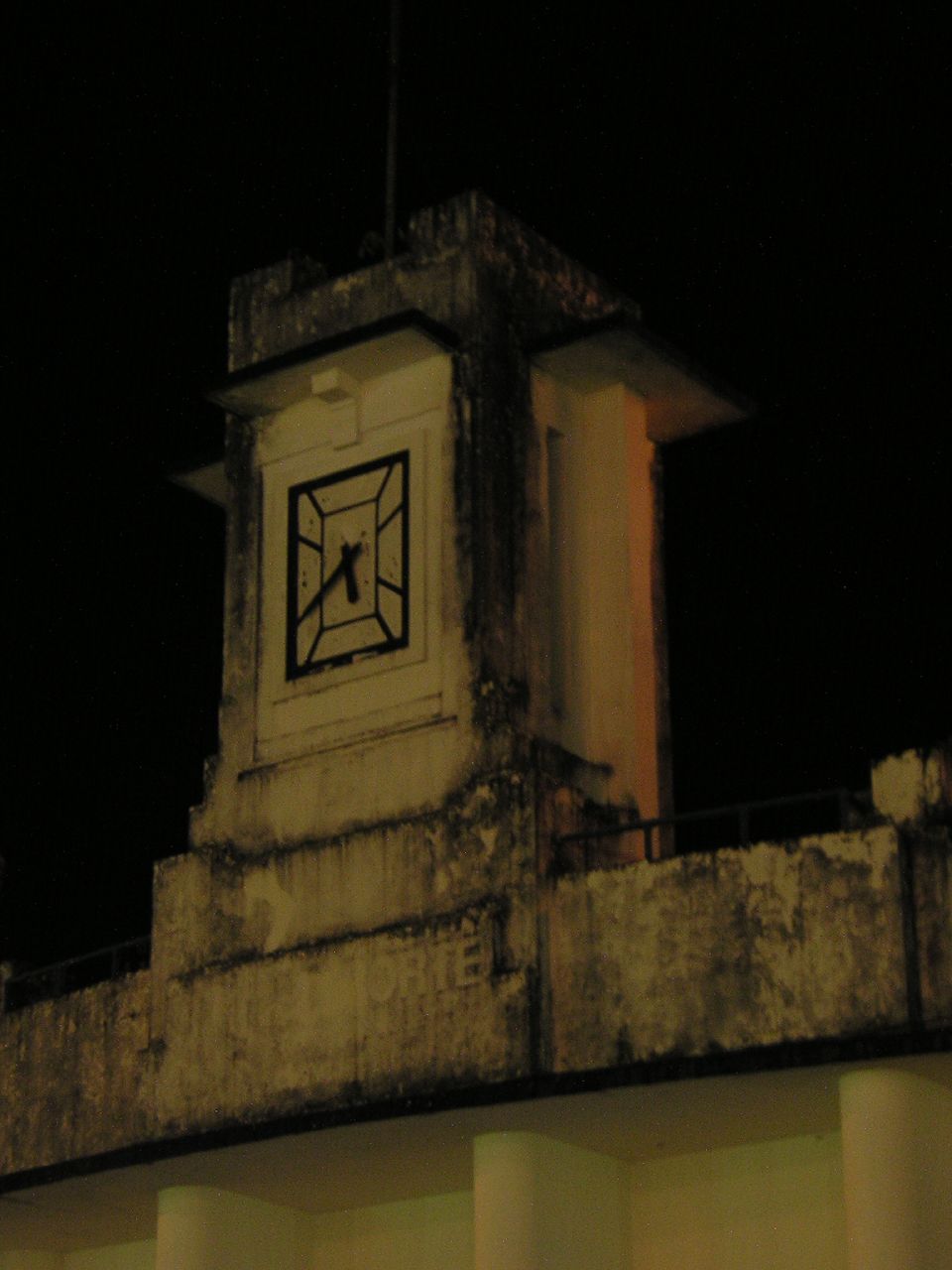This is an outdoor nighttime photograph depicting a weathered stone clock tower set against a pitch-black sky devoid of stars or moonlight. The clock tower, appearing to rest on a newer white concrete wall or bridge, features a rectangular clock face with a smaller central rectangle and radiating lines. The clock face lacks numerical markings and has two black hands indicating the time as approximately 5:40. The stone surrounding the clock is dirty and weathered, and near the bottom of the concrete base, partially legible letters ending in "ORTE" are visible.